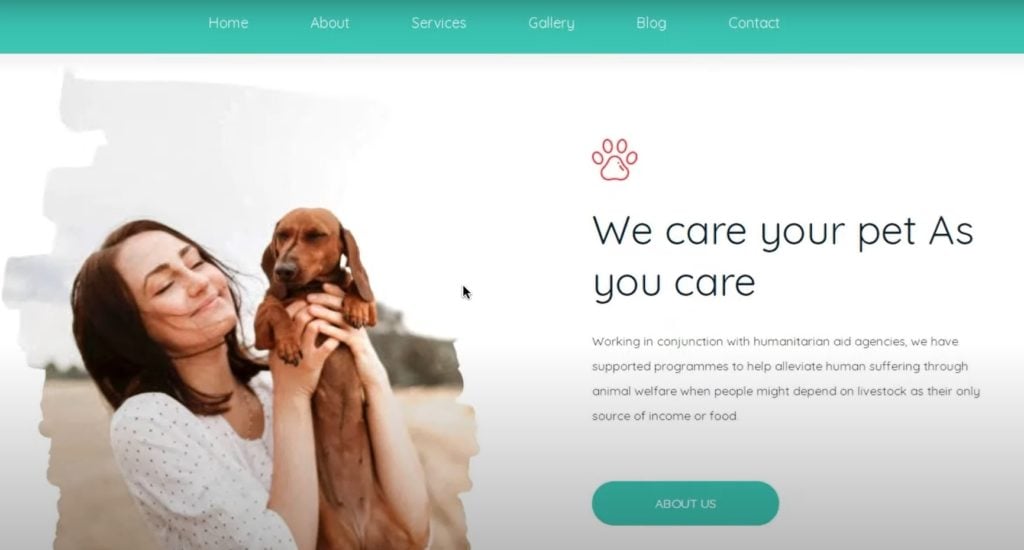Screenshot of a homepage for a pet care website: The top section features a blue menu bar with navigation options labeled Home, About, Services, Gallery, Blog, and Contact. Below, to the left, there is a visually striking photograph with torn, shredded edges. The image captures a young woman, likely in her mid-30s, standing outdoors with the wind gently blowing through her hair. She is joyfully holding up a relaxed dachshund, its belly hanging down and eyes peacefully closed. Both the woman and the dachshund are smiling, creating a heartwarming scene. To the right of the image, there's a lavender paw print icon and a somewhat awkwardly phrased tagline: "We Care Your Pet As You Care."

This section is accompanied by a brief, informative message indicating that the organization partners with humanitarian aid agencies to support programs aimed at alleviating human suffering through animal welfare. It mentions initiatives to assist communities that depend on livestock for income or food. Below this message is a teal button with the text "About Us" in white.

Notably, the design of the homepage appears to be incomplete or in progress. There is an obvious lack of branding, as the company's name is not mentioned anywhere, and important information seems to be missing. The cursor is visibly centered on the screen, suggesting that the screenshot might have been taken during the design phase. Overall, it portrays an underdeveloped and unpolished layout, which would need significant improvements before being a fully functional website.